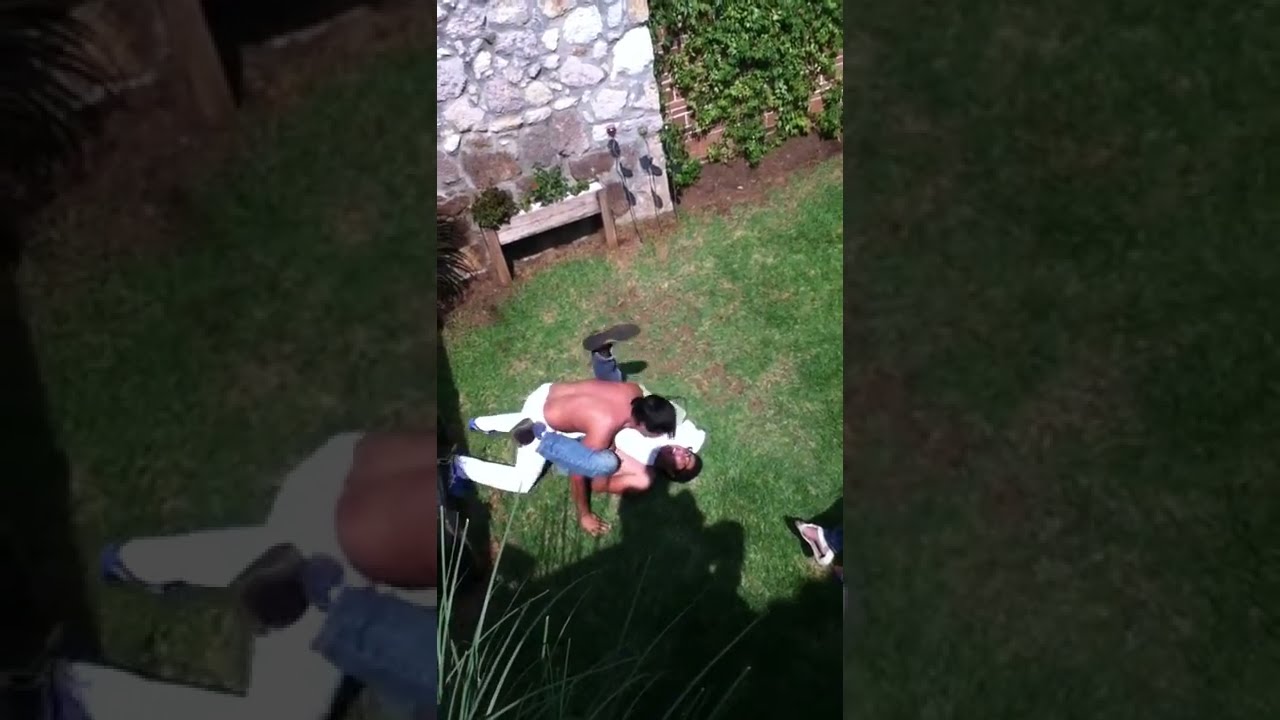In this detailed photograph, two men, both with dark hair and dark skin, engage in what appears to be a wrestling match on a grassy surface. The man on top, who is shirtless and wearing white pants, has pinned the other man, who is also shirtless but wearing blue jeans and black shoes, to the ground. Both men's positions are dynamic, with the pinned man's legs straight up on either side of his opponent. 

The scene is set outdoors and framed by various elements. In the background to the left, there is a rustic stone wall, which almost resembles a chimney but isn’t one; it features a hole at its base and consists of a series of cobblestones. Adjacent to this wall, there’s a planter box that appears to be made of wood, containing some kind of plants. To the right, another wall covered in either moss or creeping ivy is visible, enhancing the natural ambiance. Additionally, blades of grass sprout upwards in the foreground, adding texture to the scene.

In the bottom right corner of the image, the foot of another person is partially visible, and there is also some kind of shadow at the bottom of the photograph. The entire image feels encapsulated within a dark filter, drawing focus to the central action and the detailed surroundings.